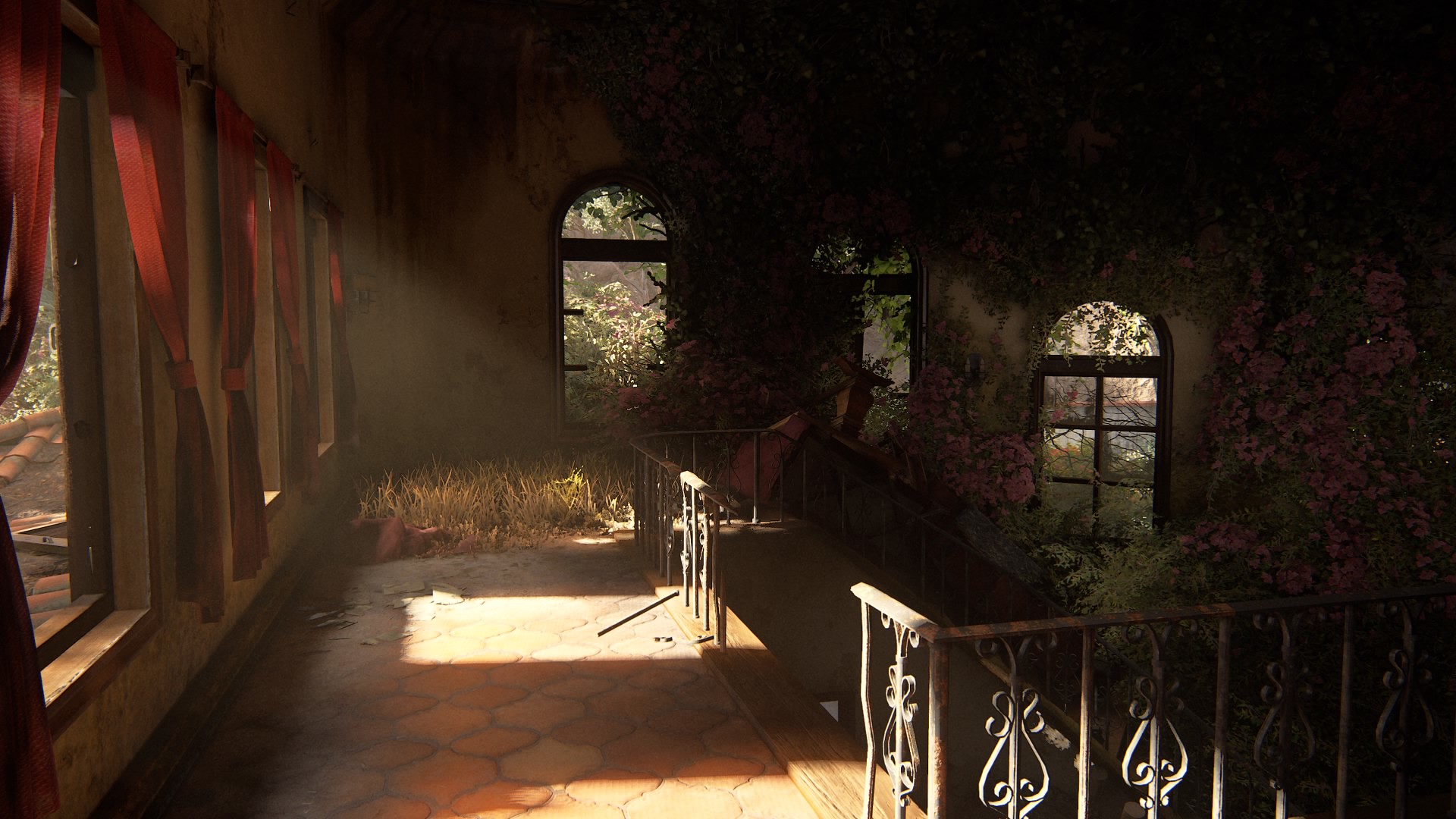The image, which appears to be a detailed color screenshot from a video game, possibly The Last of Us 2, depicts the inside of an abandoned home. The left side of the image features several wall-to-ceiling windows with red drapes pulled back, allowing an incredible amount of sunlight to cascade through the broken frames onto an empty tiled hallway. The floor consists of orange hexagonal tiles, some of which are overgrown with dead grass, suggesting long-term abandonment. On the far right, pink flowers, resembling wildly growing vines, can be seen proliferating along the wall and ceiling, adding a vibrant touch amidst the decay. An iron railing with a noticeable gap separates the walkway from the overgrown vegetation below, illuminated by streaming sunlight that casts a warm, yellow glow across the scene. This high level of detail and atmospheric lighting contribute to the haunting and desolate ambiance of the abandoned interior.